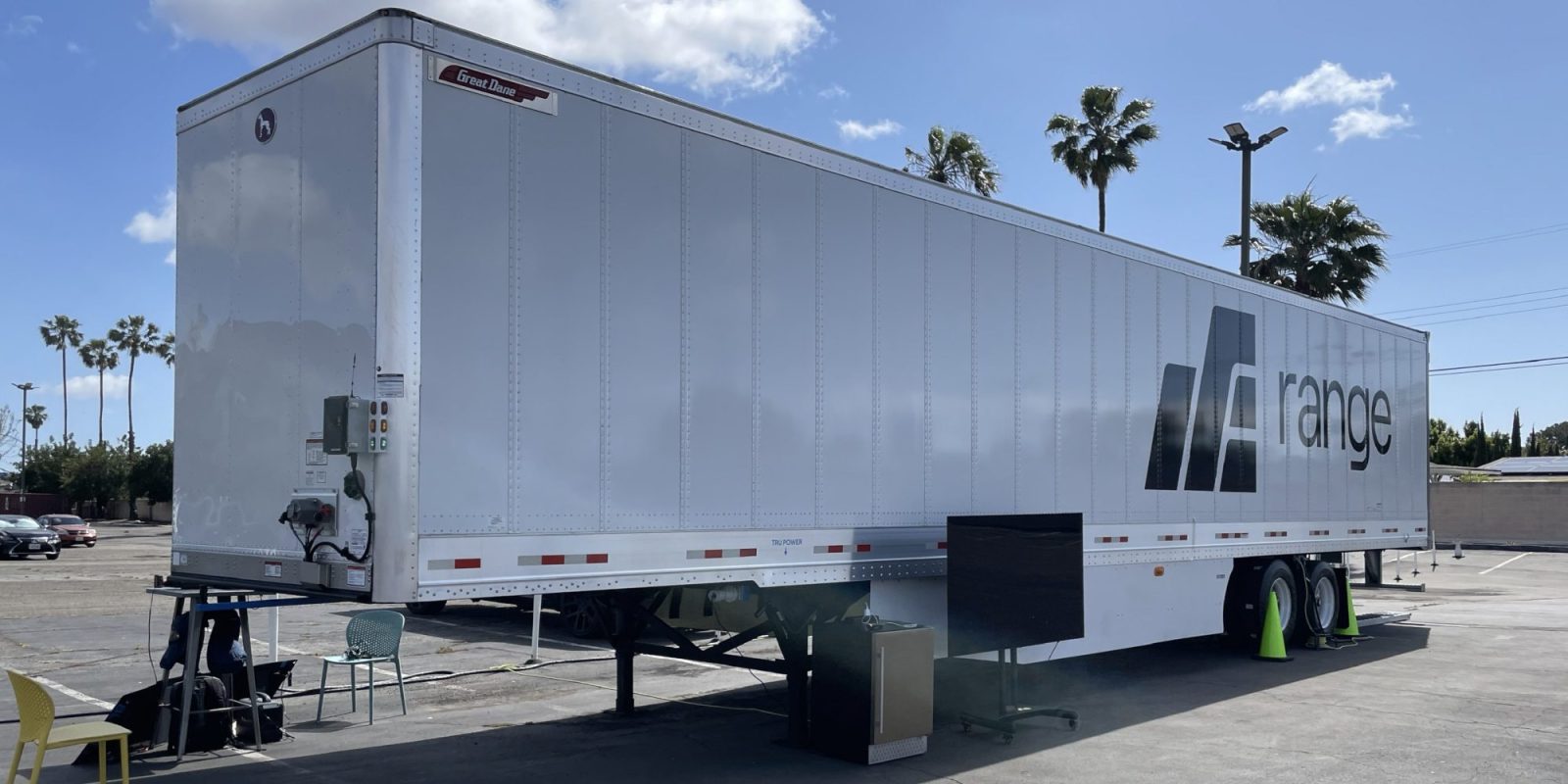The image captures a long, white tractor trailer, resembling the back of an 18-wheeler, adorned with silver trimming along its top, bottom, and corners. The trailer features a company logo towards the back right end that includes black shapes with the letter "A" inside one of them, and the word "Range" written in black on the white background. The trailer is parked in an otherwise empty asphalt parking lot, with a couple of small cars visible in the distance to the left. The scene is framed by tall palm trees and greenery in the background against a blue sky with scattered white clouds. Notably, the trailer has two visible tires at the back, propped up on various tools, indicating the absence of a cab or truck connected at the front. Additionally, the bottom left corner of the image reveals a yellow chair and a blue chair, along with a speaker, a TV, and two green cones positioned by the tires.